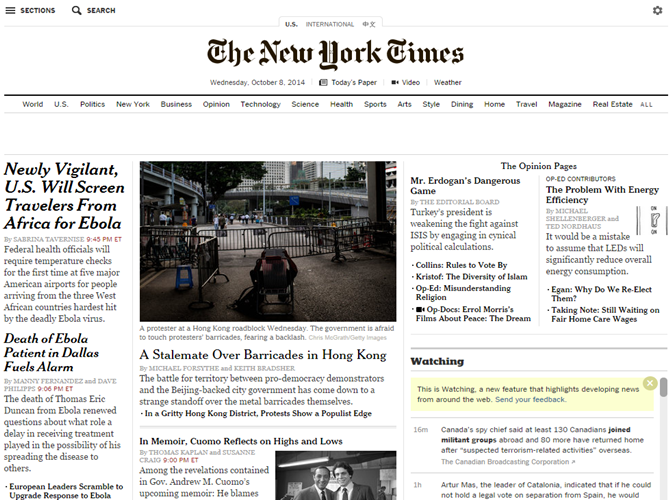**Detailed Descriptive Caption:**

The image depicts a screenshot of the New York Times website as it appeared on Wednesday, October 8, 2014. Prominently displayed at the top of the page is the New York Times logo. Above the logo, there are links for "U.S. International" news, though the third link is unclear. On the left-hand side, three horizontal lines, symbolizing a menu icon, are present next to the word "Sections". Adjacent to this is a magnifying glass icon labeled "Search". 

On the right-hand side of the top bar, a gear icon is visible, indicating settings, followed by the date: Wednesday, October 8, 2014. A series of symbols and labels follow, including an icon of a page labeled "Today's Paper," a video camera icon labeled "Video," and the word "Weather."

Below this, a horizontal black line separates the page header from the main navigation sections. The primary navigation bar includes links to various sections of the website: World, U.S., Politics, New York, Business, Opinion, Technology, Science, Health, Sports, Arts, Style, Dining, Home, Travel, Magazine, Real Estate, and an additional unclear link, possibly "All."

Featured prominently on the page is an article headline: "Newly Vigilant U.S. Will Screen Travelers from Africa for Ebola." An accompanying image shows a cityscape with numerous buildings and a fence in the foreground. Beneath this headline is another article titled "Death of Ebola Patients in Dallas Fuels Alarm."

Further down, the headline "A Statement Over Barricades in Hong Kong" is visible with a brief paragraph below. Another headline reads "In Memoir, Coma Reflects on Highs and Lows," with an image likely portraying the individual referred to as Coma and someone else. 

The section "The Opinion Pages" follows, indicating various opinion pieces with paragraphs underneath. The "Watching" section is marked by a yellow rectangle with small, unreadable text, and a green circle with an X inside it. Below "Watching," there are additional paragraphs, likely part of smaller articles or brief summaries, though the text is too small to decipher.

Overall, the website layout includes multiple navigational elements, headlines, and accompanying visual aids to provide a comprehensive news overview.